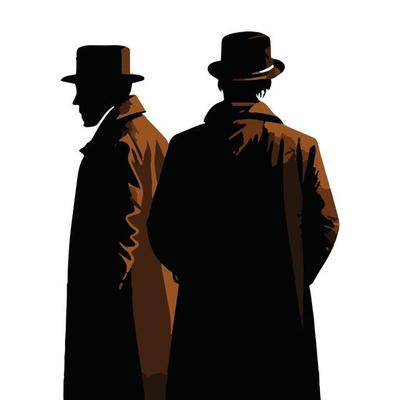A detailed graphic illustration features two mysterious male figures dressed in long, brown trench coats and brown hats, both depicted as silhouettes. Set against a white background, the image captures a moody, noir atmosphere with dramatic lighting that casts deep shadows and highlights. The man on the left, shown in profile with a flat-brimmed hat, wears a trench coat that appears lighter brown on the back due to the light and almost black in the front due to the shadows. His face is fully in shadow. The man on the right faces away from the camera, revealing only his back. His trench coat, equally darkened by shadows, hints at a light brown color on the shoulder. His hat, similar to the other man's but with a slightly tilted brim, tops shaggy hair that nearly touches his collar. Both figures exude the aura of old-school detectives, adding a touch of enigmatic elegance to the composition. The illustration is cropped to show their figures from waist up, emphasizing their iconic attire and shadowed features.